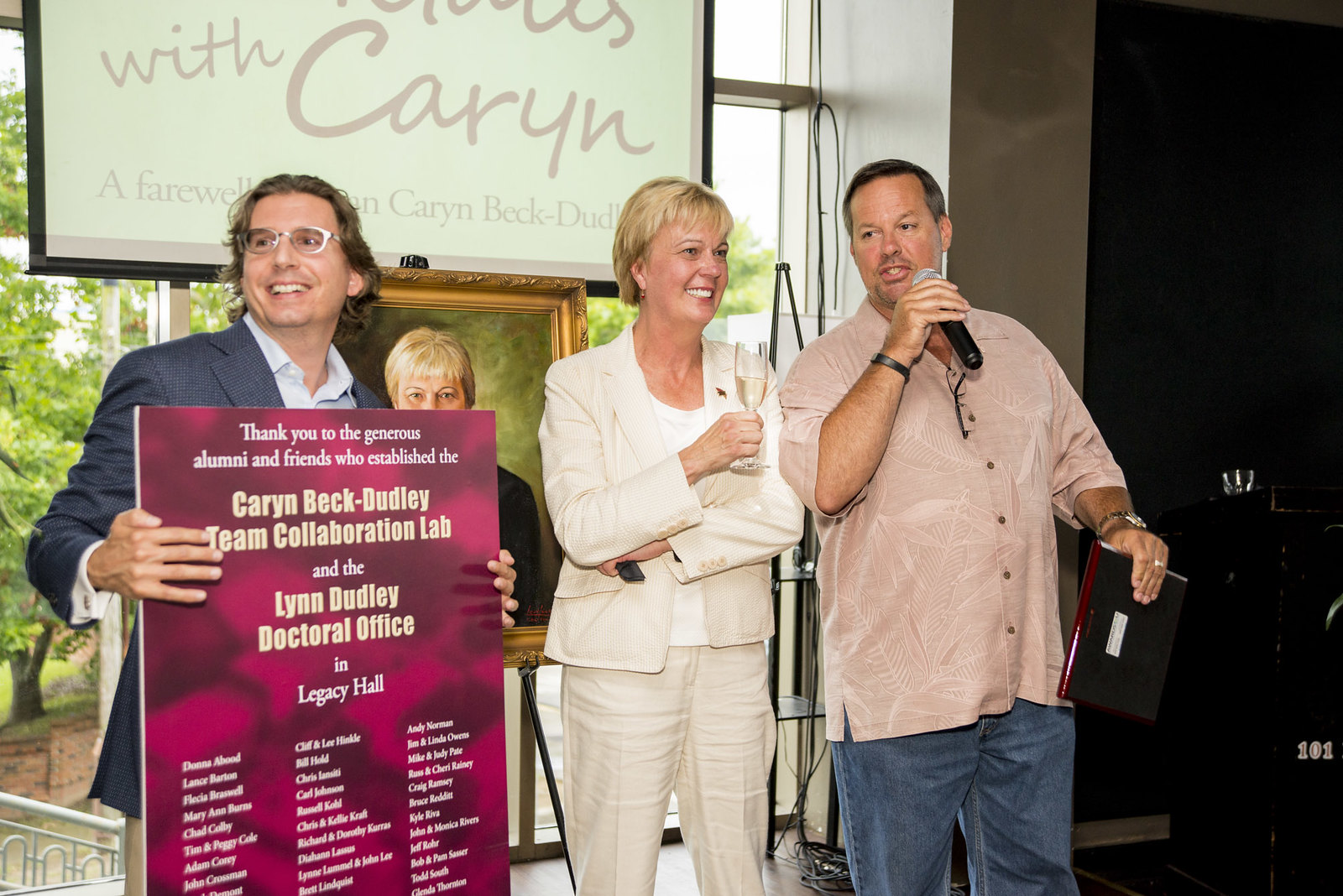In this picture, three people are standing together, seemingly at the end of a room, possibly in front of a crowd, as indicated by the presence of a microphone. The central figure is a woman dressed in a white pantsuit, holding a flute of champagne and smiling warmly. Behind her, there appears to be a portrait on an easel, featuring a woman with blonde hair and a black outfit, set against a green background, which matches her appearance, suggesting it is a painting of her.

To the woman's right is a man with slightly long, shoulder-length hair, glasses, and a blue suit paired with a blue button-down shirt. He holds a sign that reads, "Thank you to the generous alumni and friends who established the Karen Beck Dudley Team Collaboration Lab and the Lynn Dudley Doctoral Office in Legacy Hall." The sign is pink with the text centered at the top, and underneath, there appears to be a list of donors.

On the woman's left is another man, who is speaking into a microphone. He is dressed in a pink button-up shirt and jeans and holds a microphone near his mouth with his right hand and a folder with his left. This scene suggests a celebration or an event honoring the woman, likely named Karen, given the references on the sign and in the portrait behind her.